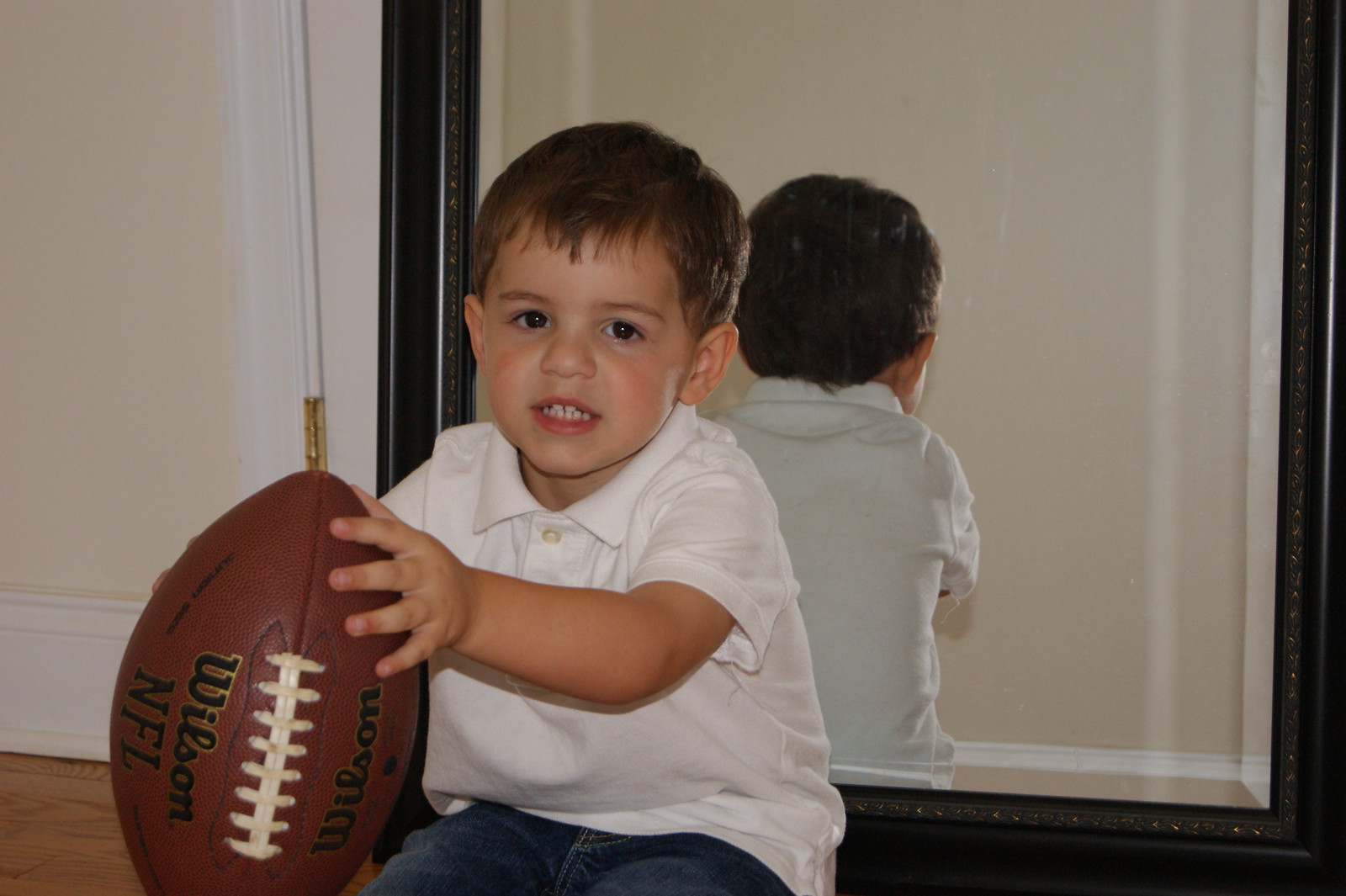In the picture, a young boy, approximately two to three years old, is seated on the brown hardwood floor. He is wearing a white button-down polo shirt and blue jeans. The boy has short brown hair with some strands falling over his forehead and light eyes. He is holding a regulation-size Wilson NFL football with both hands, showcasing its white laces and black branding towards the camera. His cheerful expression reveals a full, but slightly strained, smile beneath his red cheeks.

The child is positioned in front of a tall, black-framed mirror, which reflects the back of his head and the room's white walls. The mirror's reflection also reveals a door to his left, highlighted by gold hinges and a white trim. This additional perspective adds depth to the scene, emphasizing the boy's joy as he grips the oversized football.